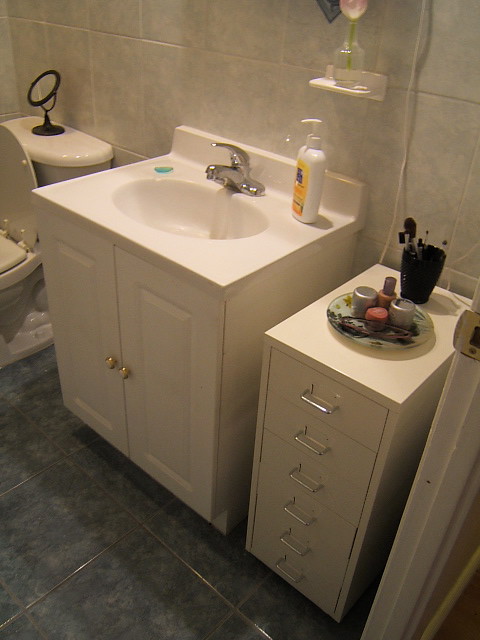This photograph captures a well-organized bathroom vanity area with intricate details. Dominating the center, a white vanity is elegantly enhanced by a chrome-colored faucet and a soap dispenser bearing a yellow label. To the far left in the background, a toilet is visible with its black mirror resting on the tank and the seat notably up. 

Adjacent to the vanity on the right stands a set of six drawers, crowned with a glass plate that holds an assortment of makeup items, a candle, and a pair of glasses. Right behind this setup, a black cup is filled with what appear to be makeup brushes or possibly shaving tools. Beyond this display is a small gap revealing the doorway where the photographer is positioned, discernible by the door latch mechanism.

The bathroom’s ambiance is completed by a backdrop of white-tiled walls with distinct grout lines, and underfoot, a textured grayish tile floor with contrasting darker grout. Every element combines to provide a comprehensive and meticulously detailed view of this bathroom corner.